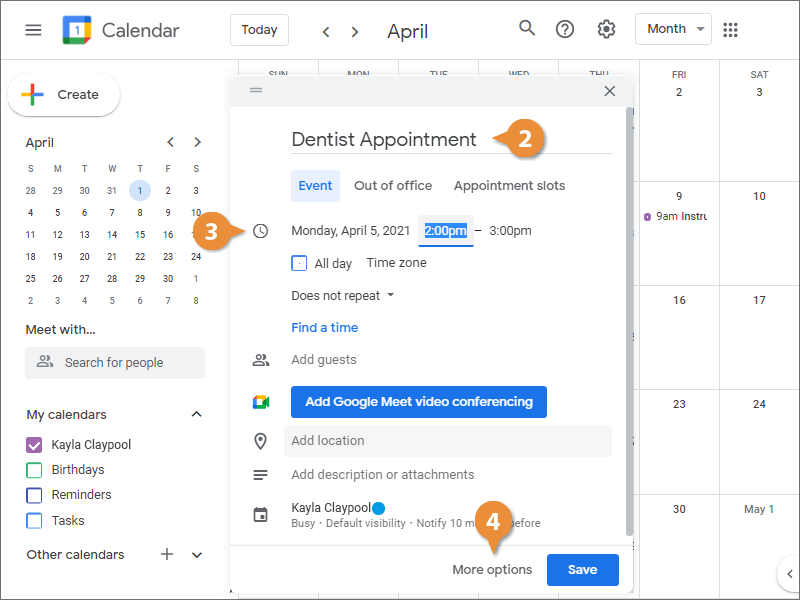A detailed screenshot of a Google Calendar page displayed on a laptop, showcasing an intricate tutorial. In the foreground, a pop-up detailing a dentist appointment is prominently visible. The appointment is scheduled for April 5th, 2021, at 2 p.m., with the location information clearly displayed. Surrounding the pop-up, large dark orange bubble highlights are numbered, indicating steps in a tutorial likely explaining various features or actions within the calendar.

In the background, the typical day-by-day view of the April calendar can be partially seen, though mostly obscured by the appointment pop-up. To the left, a mini April calendar is present, showing dates without the usual squares, allowing for a general overview of scheduled events. 

Below the mini calendar, the "My Calendars" section lists four different calendars: "Kayla's Clay Pool," "Birthdays," "Reminders," and "Tasks," with only "Kayla's Clay Pool" selected, meaning only appointments from this calendar are displayed.

This detailed image reflects the organized interface of Google Calendar, enhanced by an educational overlay for better user understanding.